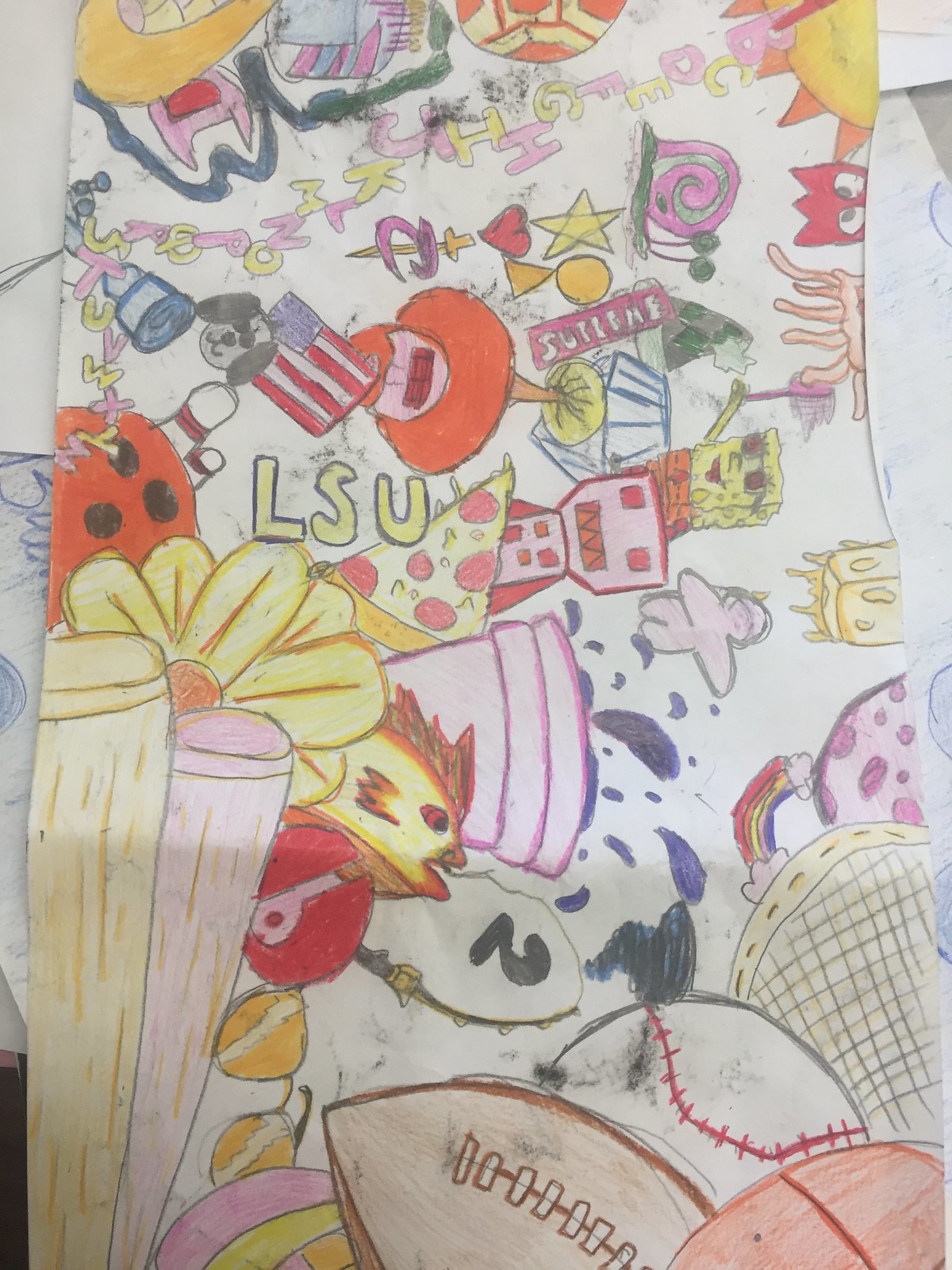In the center of a diverse collage on paper, various sports items and other miscellaneous objects are prominently displayed. At the bottom, there's a brown football. Above it, a white baseball with distinct red stitches is shown. Nearby, a colorful scene includes an athlete and what appears to be a rainbow alongside a purple flower vase with water sprouting out of it. To the left, a bouquet featuring yellow and purple coneflowers is seen, with a yellow flower situated behind them. There is also an ambiguously shaped figure resembling either a fish or a chicken with a red hood. 

On the left-hand side, a dark bowling ball is positioned next to a set of upright bowling pins in the background. The LSU logo is visible in the mix, accompanied by illustrations of pizza, a robot, and a character that resembles Spongebob Squarepants, although the figure appears to be a child. Behind what looks like a tooth, a red egg bearing the "Supreme" logo is displayed. Along the top of the image, an alphabet string runs across, concluding with a sign at the top right corner.